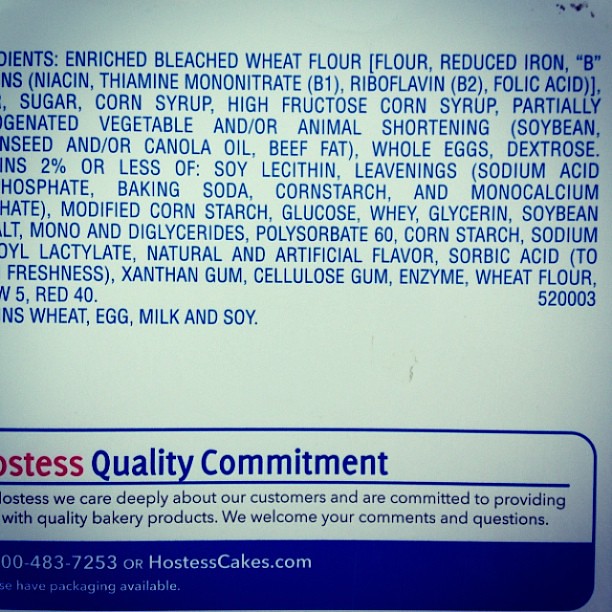**Descriptive Caption:**
The image features a white ingredients label on the back of a food product container, with all the text printed in blue letters. Despite parts of the writing being cut off in the picture, you can still read most of the listed ingredients. The partial list includes: enriched bleach, wheat flour, reduced iron, niacin, thiamine mononitrate (B1), riboflavin (B2), folic acid, sugar, corn syrup, high fructose corn syrup, partially hydrogenated vegetable and/or animal shortening (soybean and/or canola oil), beef fat, whole eggs, dextrose, soy lecithin, leavening agents (sodium acid pyrophosphate, baking soda, monocalcium phosphate), modified corn starch, glucose, whey, glycerin, soybean mono and diglycerides, polysorbate 60, sodium stearoyl lactylate, natural and artificial flavors, sorbic acid (for freshness), xanthan gum, cellulose gum, enzymes, and Red 40. The label also includes allergy information, indicating the presence of wheat, eggs, milk, and soy.